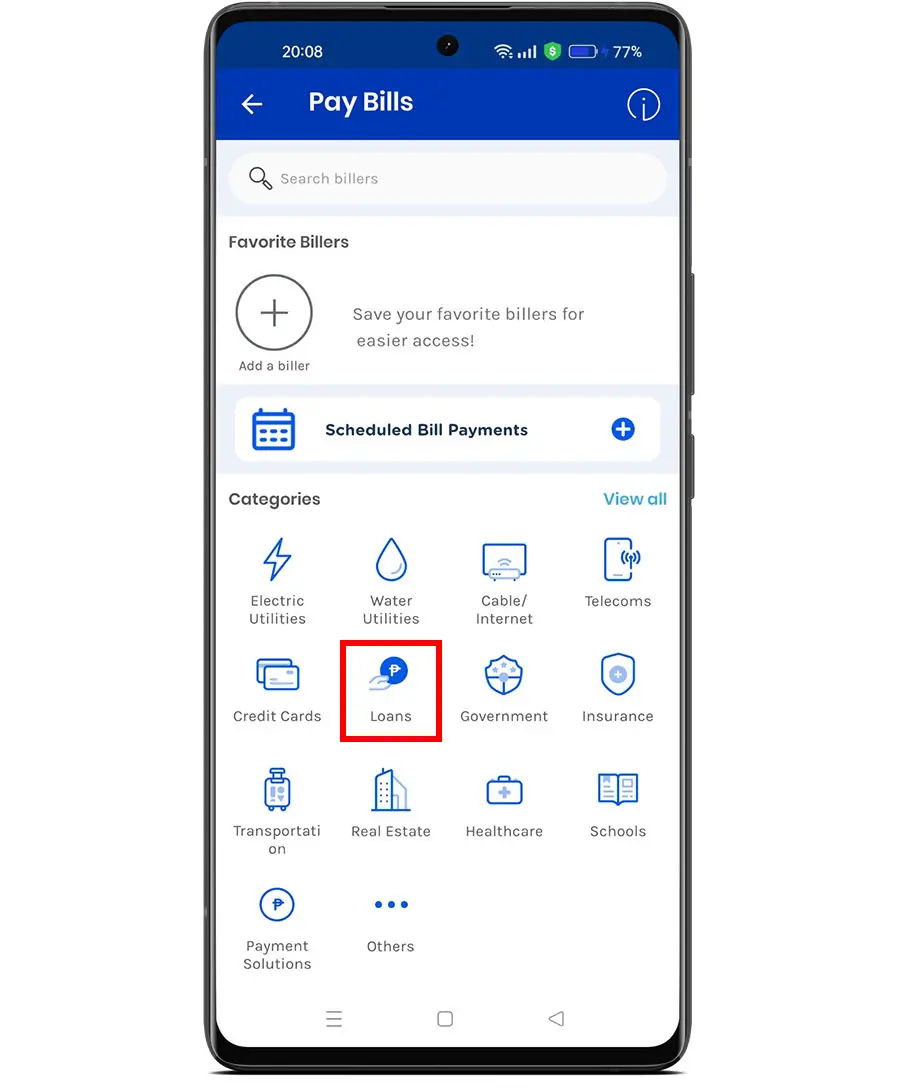This image is a detailed screenshot of a smartphone screen, displaying a bill payment app interface. The entire phone is visible, revealing the current time on the top left corner and various status icons, such as battery percentage, on the top right.

In the upper section of the screen, there is a prominent blue header with the label "Pay Bills." To the left of this label is a white left-pointing arrow, and to its right, there is an eye-shaped icon.

Below this header, the interface transitions to a white background. At the top of this section is a search bar labeled "Search Billers." Directly beneath the search bar, there is a section titled "Favorite Billers." Within this section, there is a plus icon enclosed in a circle with the text "Add a Biller" beside it. To the right of this, a note reads, "Save your favorite billers for easier access."

Further down the screen, there's a segment indicating "Scheduled Bill Payments" accompanied by a calendar icon and a plus symbol. Immediately following this, there is a "Categories" section with a "View All" option to its right.

Within the categories section, a variety of bill types are organized with corresponding icons:
- Electric Utilities: Represented by a lightning bolt icon.
- Water Utilities: Illustrated with a water droplet icon.
- Cable Internet
- Telecoms
- Credit Cards
- Loans: Highlighted with a red square around its label.
- Government
- Insurance
- Transportation
- Real Estate
- Health Care: Represented with a suitcase icon.
- Schools
- Payment Solutions
- Others

Each category has a unique symbol representing the type of service, providing a visual cue for users to quickly identify their specific billing choices.